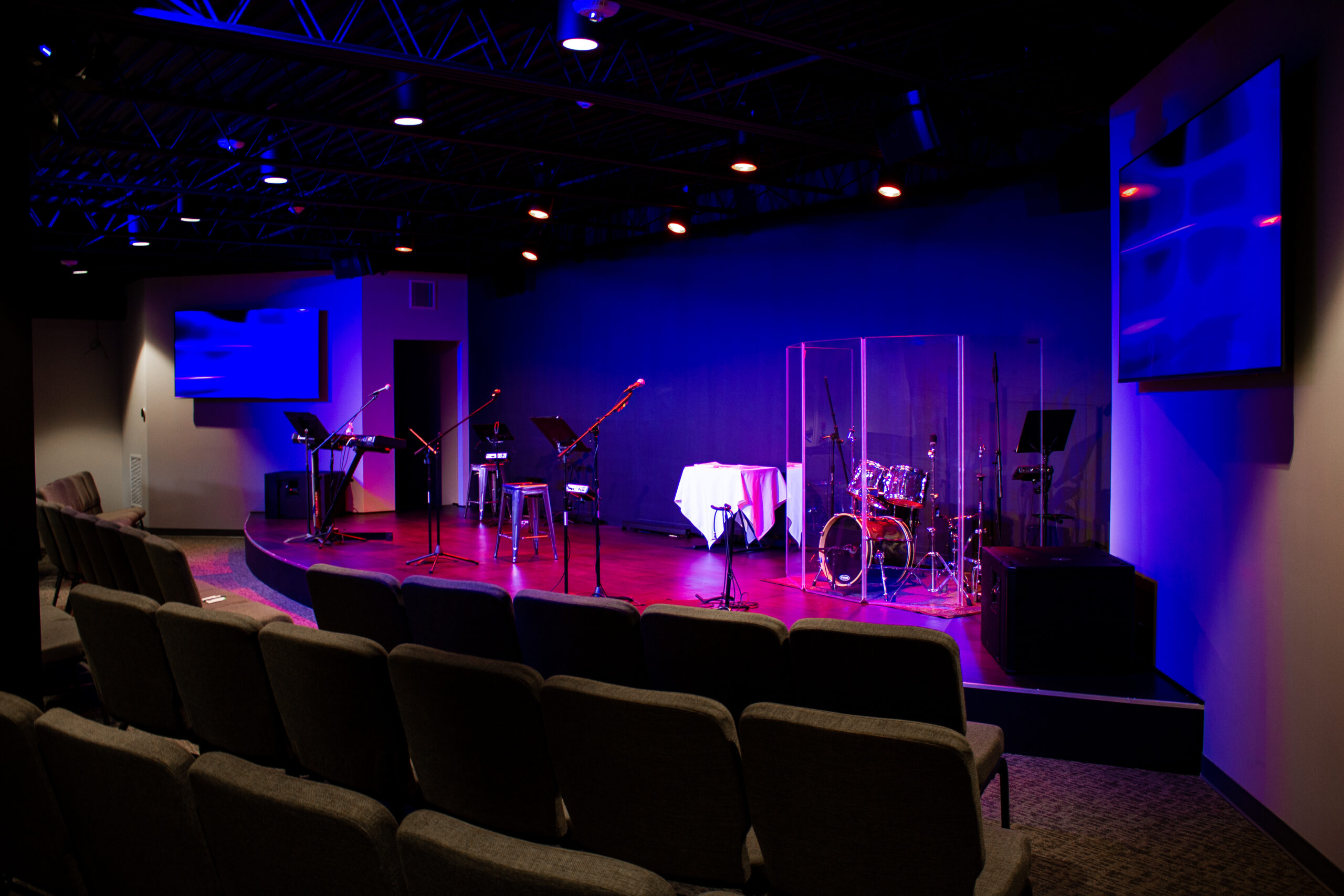The photograph depicts an empty concert studio that appears intimate and compact. The perspective is from about four rows back on the right-hand side, looking onto the stage. The foreground showcases three rows of flat theater seats that span from the left-middle of the image to the right side; these seats are gray. Beyond the seating area, the stage is set up, featuring a drum set enclosed behind glass likely for sound muting. The stage floor is illuminated with a pink light, contrasting with the blue backdrop, creating a vibrant, nightclub-like atmosphere in the otherwise dark room. A table draped in a white tablecloth is positioned adjacent to the drums. Besides the table, there are three microphone stands and a stool with a red top. Further to the left, there's a keyboard setup. The lighting setup includes spotlights arranged in three rows overhead, casting focused illumination on both the stage and the area just before it. Large TV screens are mounted to the far left of the stage and to the right, possibly intended for advertisements or live video feeds of the performance. The overall scene is carefully staged for a concert, yet remains void of any audience or performers.